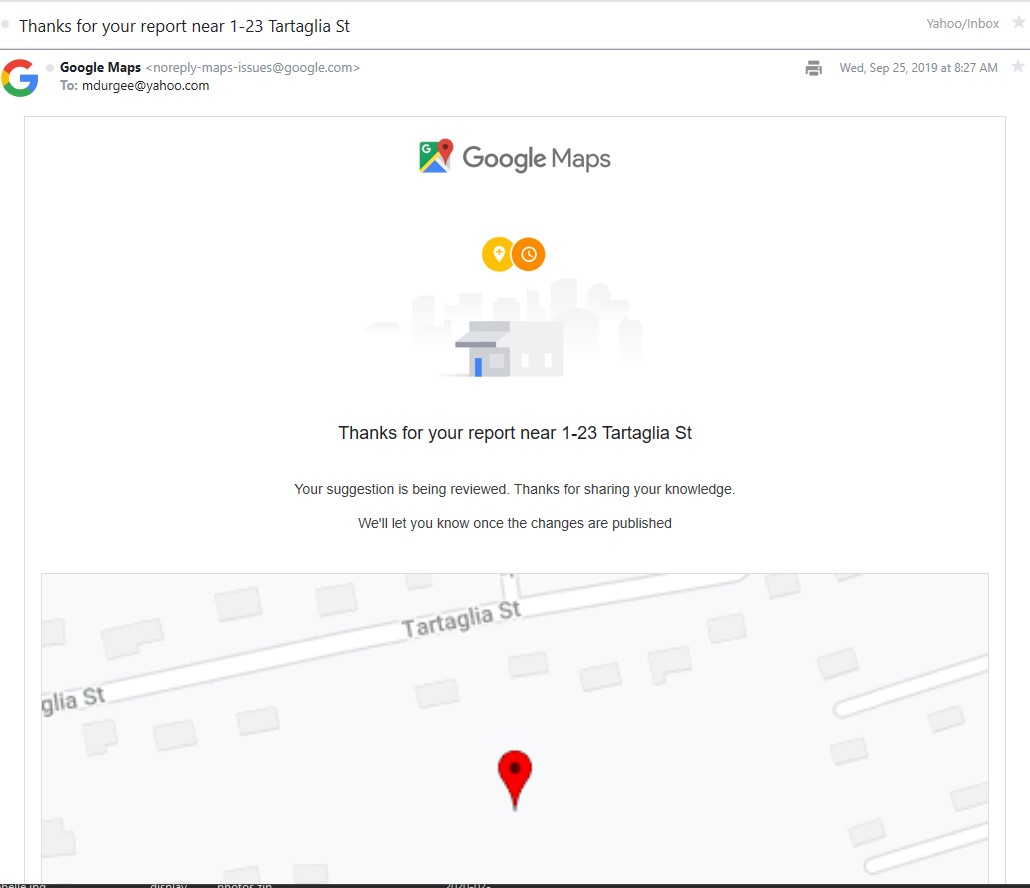This is a detailed screenshot of an email received from Google Maps, displayed in a web browser. The email header confirms that it is from a no-reply address at Google Maps (no-reply-maps-issues@google.com), and it was sent on Wednesday, September 25th, 2019, at 8:27 a.m. The recipient is identified as mdurgee at a Yahoo email address (mdurgee@yahoo.com). The subject matter of the email pertains to a report made near 1-23 Tartaglia Street.

The email begins with the Google Maps logo and a courteous acknowledgment: "Thanks for your report near 1-23 Tartaglia Street." The main content informs the user that their suggestion is under review and expresses gratitude for their contribution. The email also assures the recipient that they will be notified once any changes are implemented.

A small map embedded within the email displays a close-up of Tartaglia Street, marked with a red locator arrow, pinpointing the specific location in question. On the right side of the screenshot, there is a visible browser tab label, "Yahoo/Inbox," indicating that the email is being viewed within a Yahoo Mail interface.